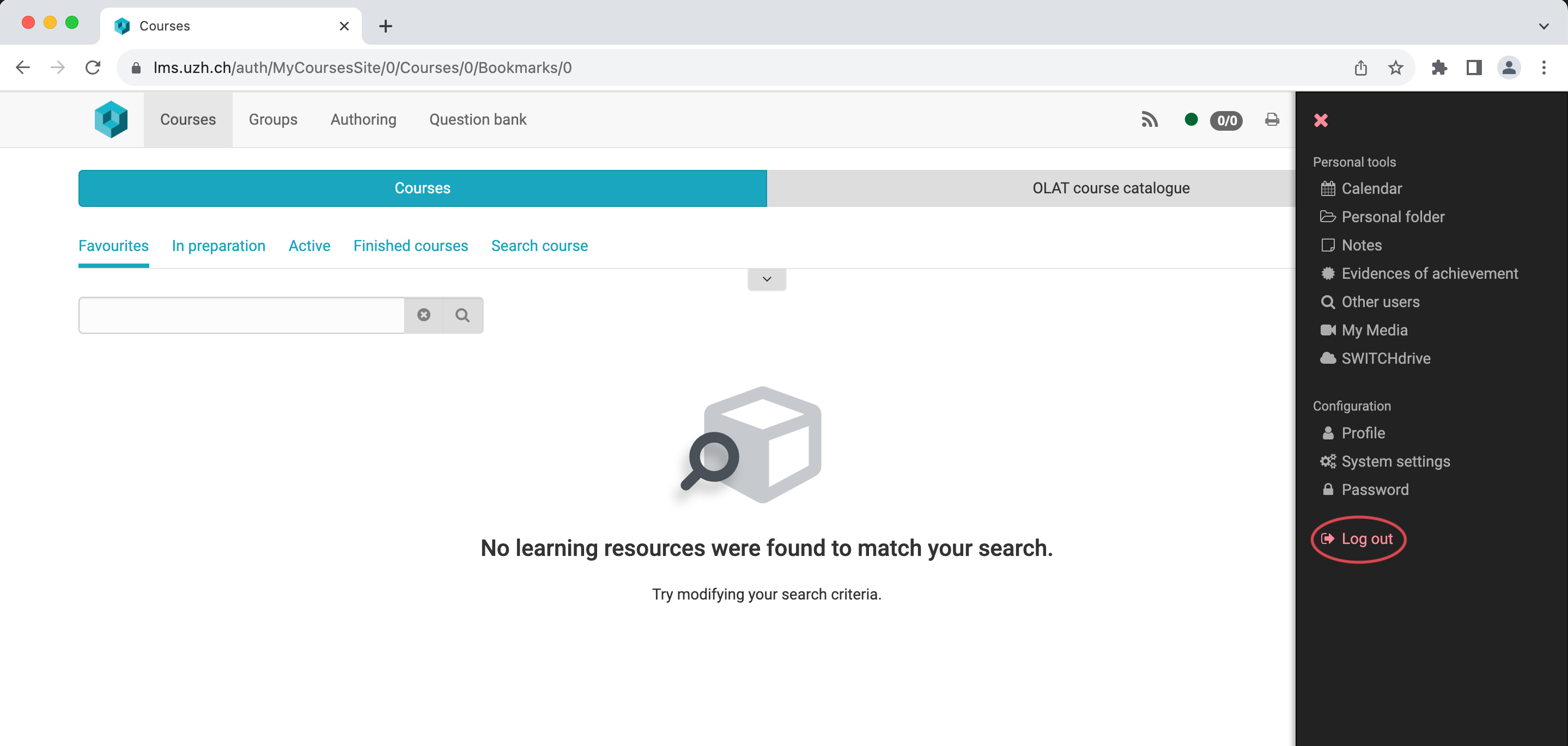The image showcases a comprehensive webpage that serves as a dashboard for various educational tools and resources. At the top, the navigation bar includes options such as Courses, Groups, Authoring, Question Bank, Favorites, Preparation, Active Courses, Finished Courses, and a Search Course feature. Below these tabs, a prominent search bar is visible with a magnifying glass icon on its right side, facilitating quick searches for courses.

On the right side of the page, there is a dropdown menu providing access to an array of personal tools and settings. These include Calendar, Personal Folder, Notes, Evidence of Achievements, Other Users, My Media, Switch, Drive, Configuration, Profile, System Settings, Password, and Logout features.

The webpage is intuitively designed to support institutional work, offering a centralized platform for educational management. The layout indicates that the site is tailored to accommodate a diverse user base, facilitating efficient access to various educational and administrative resources.